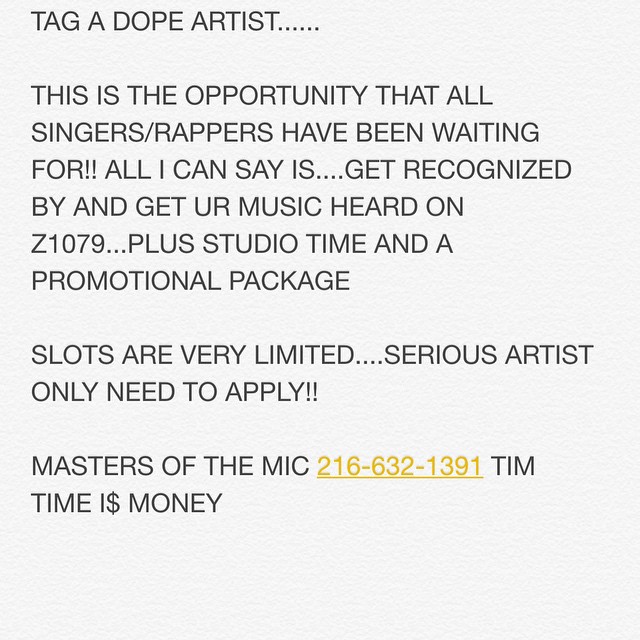The image is entirely text-based, featuring black text on a white background with the phone number in gold and underlined. The advertisement reads from top to bottom: "TAG A DOPE ARTIST..." followed by a new paragraph stating, "This is the opportunity that all singers/rappers have been waiting for!! All I can say is... get recognized by and get your music heard on Z1079... plus studio time and a promotional package." Another paragraph follows with, "Slots are very limited... serious artists only need apply!! Masters of the mic." It concludes with the contact information: "216-632-1391, Tim." Highlighting the urgency, the text ends with, "Time is money" where the "S" in "is" is replaced by a dollar sign.